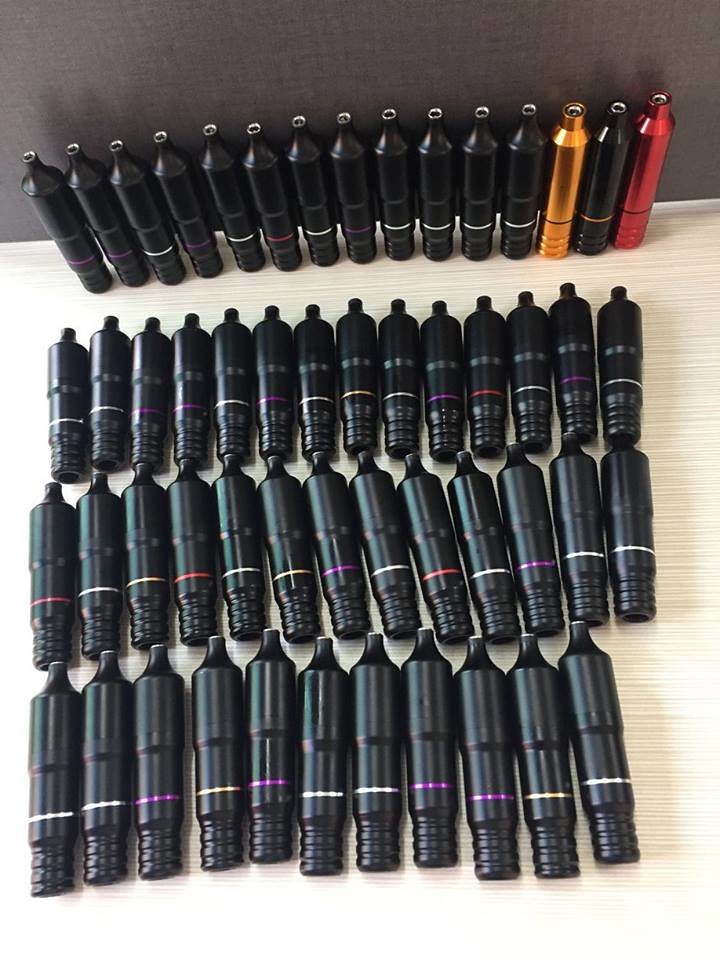This indoor scene captures a collection of conical canisters arranged on a pale, likely hardwood or light beige surface, possibly serving as a floor or table. The setup includes four rows of these bottle-like objects. Three of these rows lie horizontally, while the back row stands upright against a dark gray wall. Most of the canisters are black, but distinctively, the upright row includes an orange canister, a red one, and several black ones. The black canisters feature a colored band around them near their screw-in bottoms, with variations of red, purple, yellow, white, and silver accents. The conical canisters have narrow bases and small silver openings at the top, resembling water bottles but with a distinct design suggesting they might be designed to be screwed into something. The photograph is rectangular, providing a clear and comprehensive view of the entire arrangement.